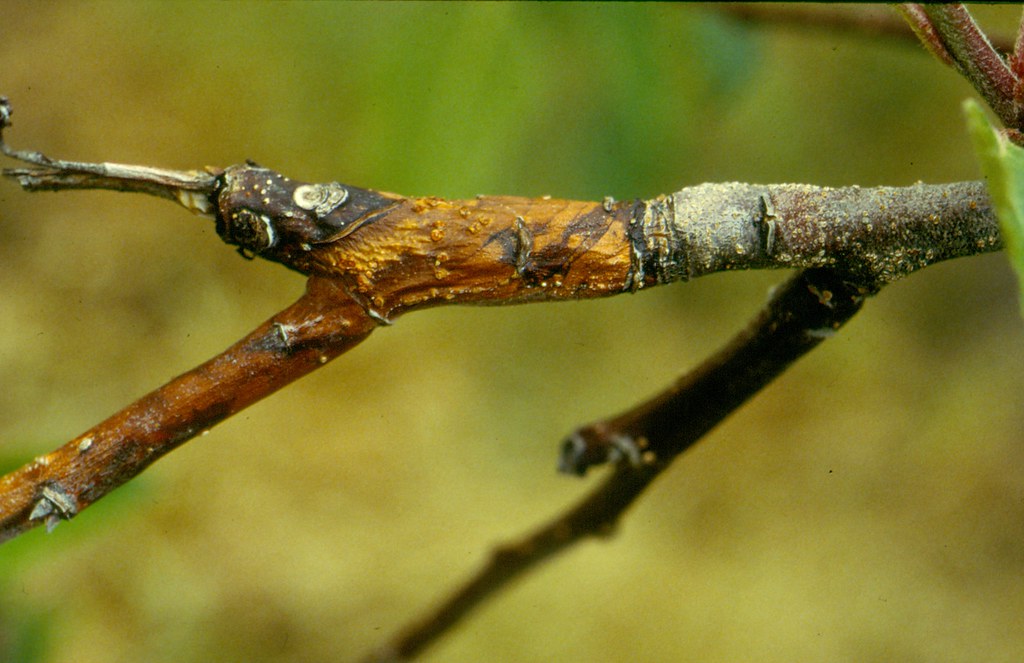This close-up macro photograph captures an intricately camouflaged walking stick insect blending seamlessly with its forest environment. The insect's elongated body and legs mimic the appearance of tree branches, exhibiting a brown coloration speckled with white spots resembling mold growth. Detailed features such as its eyes and head are visible, further adorned with the same brown and white pattern, enhancing its deceptive disguise. The background is a blurred mix of green and brown hues, suggesting a lush forest setting where this master of disguise was discovered. Incredibly, the bug's mimicry is so convincing that at first glance, one might easily mistake it for an ordinary tree branch adorned with mold.